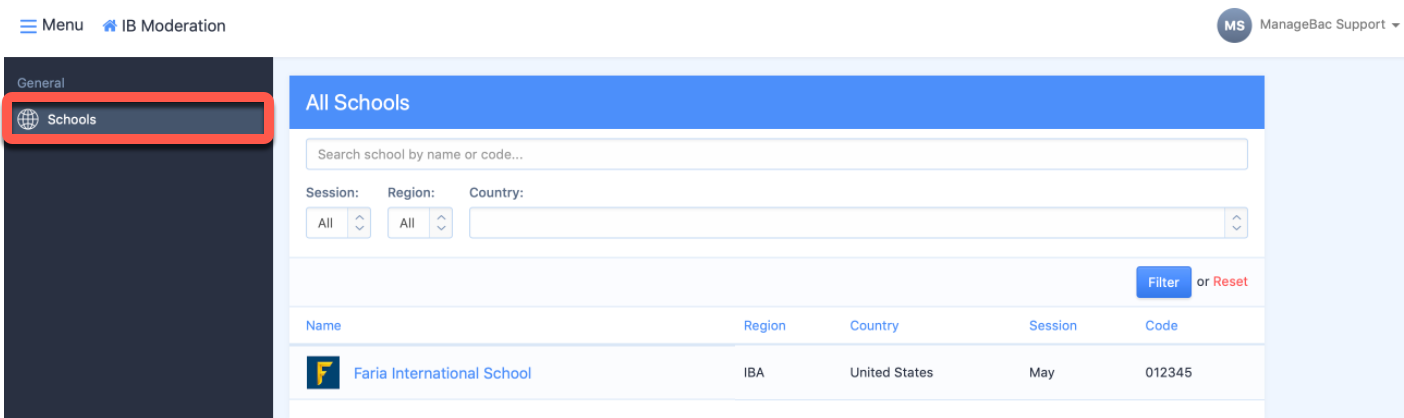Here is a detailed caption for the given screenshot:

This image showcases a screenshot of an educational platform, capturing its user interface in detail. At the very top, a white header spans the width of the screen. On the far left of this header are three horizontally stacked blue lines, which constitute the menu icon, accompanied by black text that reads "Menu." Adjacent to this, to the right, is a blue house icon followed by the black text "IB Moderation."

In the top right corner of the white header, there is a gray circle containing the white initials "MS." Directly next to this, the medium gray text "Manage Back Support" is displayed, with a downward-pointing arrow indicating a dropdown menu.

To the left of the main body of the page, a dark gray sidebar is present. At the top left of the sidebar, light gray text reads "General." Beneath this label, a medium gray rectangle features a white globe icon on the left, accompanied by the white text "Schools." This rectangle is highlighted by a red outline, signifying its active status.

The main content area of the page lies to the right of the sidebar and is framed by a light blue background. Positioned on this background is a central white rectangle. At the top of this white section, a medium blue header contains the white text "All Schools" aligned to the left.

Below this blue header, a white search box is situated, inside of which light gray placeholder text reads "Search School by Name or Code." Further down are three dropdown menus, each labeled with bold text. The first dropdown is labeled "Session," containing the text "All" and flanked by an up-and-down double arrow. The second, to its right, is labeled "Region" and similarly displays "All" with double arrows. The third dropdown, which is longer than the previous two, is labeled "Country" and also features the double arrows. 

Beneath this set of dropdown menus is another section, though it is not fully visible in the screenshot.